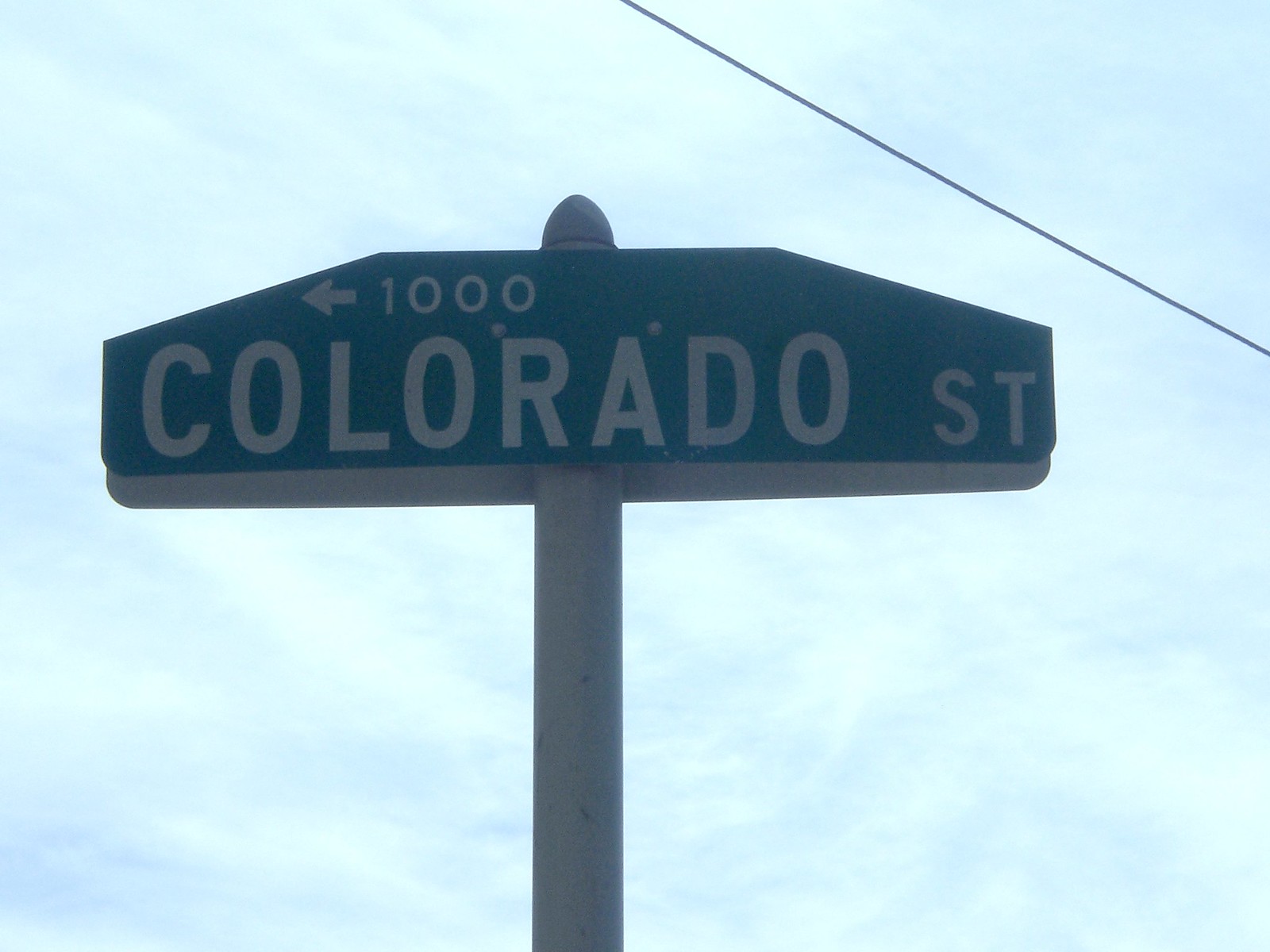This image showcases a green street sign mounted on a silver pole, set against a very light blue sky adorned with some white clouds. The street sign has a flat bottom with slightly raised sides, culminating in a rounded top. In pristine white letters, the sign prominently displays the number "1,000" and, below that in larger, bolded letters, the name "Colorado" with the abbreviation "ST" for street. A black line descends from the top center of the image, extending diagonally to the right side, adding an element of intrigue to the otherwise serene sky.